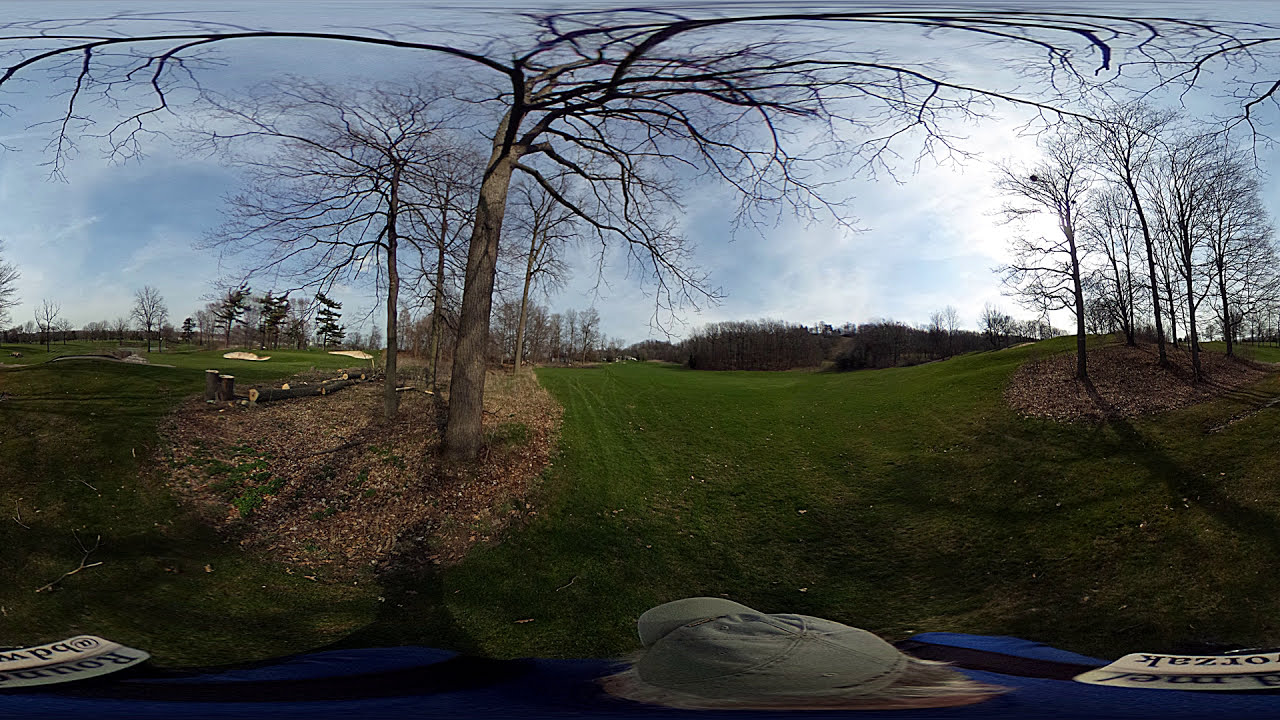The panoramic image, taken with a fish-eye lens, captures a sweeping outdoor landscape. The bottom portion of the image is marked by a strip of distorted visuals, including an upside-down sign with the partially legible words "O-R-Z-A-K" and "R-O-U-N B-D-W@", and what seems to be a distorted gray baseball cap and some blond hair. In the middle, there is a mix of vivid green grass and patches covered in dead leaves, with clusters of bare trees. To the right, more bare trees arise from a leaf-strewn ground. In the far background, beyond the main grouping of trees, lies a golf course with identifiable sand traps and various scattered logs and stumps. The horizon is lined with more trees, some of which have a few leaves. The sky above is overcast, blending patches of blue with prevalent white clouds, and a bright area on the right possibly hiding the sun.